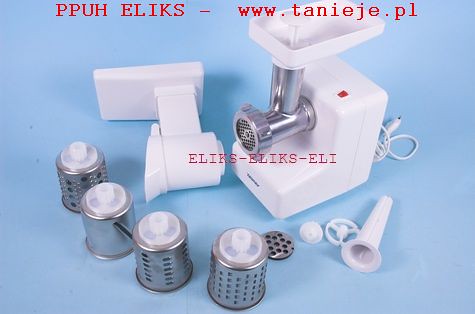This image showcases a sleek, white, electric kitchen appliance, primarily designed for grinding or juicing with versatile functionality. The equipment features a white plastic body accentuated with key metal components, including a silver grinding tube with a metal grate at the front. Attached to the main unit via a visible cord is a red on/off button. The appliance includes a white platform where ingredients can be inserted into the metal tube, complemented by a plunger to facilitate the process. 

Furthermore, the device comes with four distinct metal attachments, resembling thimbles, which appear to offer various grinding settings from fine to coarse, suitable for a range of uses such as juicing, pulping, or grinding spices. There's also a thin plastic funnel and an extension piece that can be fitted onto the top of the metal pipe to modify its function. The backdrop of the photo is a soft white with a bluish hue, emphasizing the clean and modern design of the appliance. An inscription on the device reads "ppuhelix-www.tannyje.pl," indicating the manufacturer.